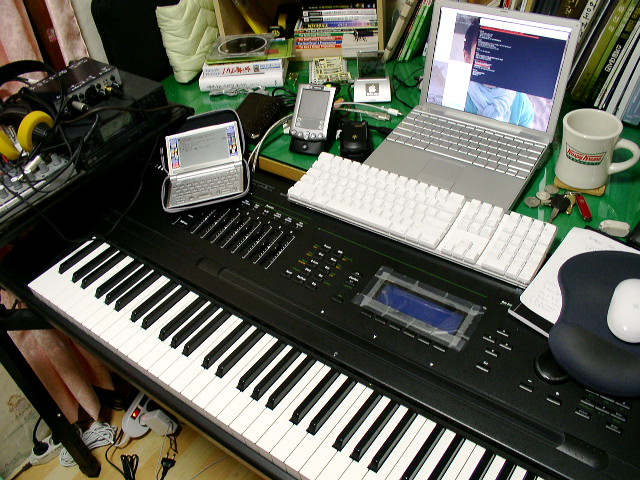A highly detailed image captures a retro music recording setup that's stationed atop an electric keyboard. The centerpiece is a silver laptop with an open text document or possibly an image of a person in a blue sweater on its screen. Just below and beside the laptop on the keyboard's surface, there are various electronic devices including a Palm Pilot and a Game Boy, suggesting a vintage aesthetic from the late 90s to early 2000s.

The workspace features a full, standalone keyboard and a white mouse, which rests on a black mouse pad with a wrist rest, indicating the user opts not to use the laptop's built-in keyboard and trackpad. To the side of these components are some yellow foam-cushioned headphones, signaling perhaps a music production or recording endeavor, supported by additional unidentified electronic devices with knobs for sound adjustments.

A Krispy Kreme coffee cup is prominently placed, among some scattered coins, keys, and a Swiss Army knife, adding to the cluttered yet functional environment. The entire setup rests on a glass tabletop with a glossy green tint. In the backdrop, there are several books adorned with East Asian script—possibly Chinese, Korean, or Japanese—enhancing the cultural impression of the space. The overall feel is one of a high-tech music production space, but one that reflects the technology and aesthetics of several decades ago.